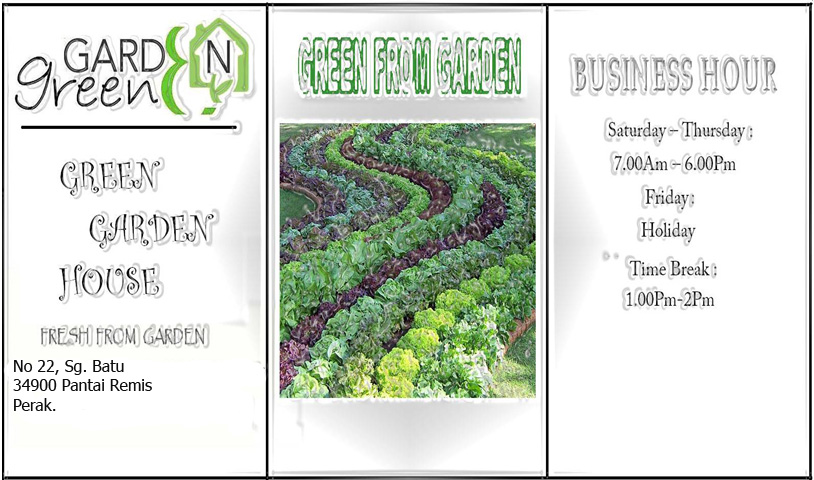The image is horizontally oriented with a white background and divided into three vertical sections outlined in black. The first section on the left features the words "Garden Green" in green text alongside a logo with the letter 'N' stylishly inside a greenhouse shape. Below this, it reads "Green Garden House, Fresh From Garden" and provides an address: "No. 22 SG Batu 34900 Pantai Remus Perak."

The central section displays the text "Green From Garden" in green, above a photograph of a garden filled with what appears to be cabbages or another type of vegetable, arranged in a distinctive snake-shaped row that curves from top to bottom. This photograph is somewhat distorted due to a plasticky Photoshop filter that overlays the entire image.

In the rightmost section, the business hours are clearly listed: "Saturday to Thursday, 7 a.m. to 6 p.m.," noting that Friday is a holiday with a time break from 1 p.m. to 2 p.m. Despite the plasticky filter making parts of the image hard to read, the overall design conveys a mix of green themes, garden produce, and business information.